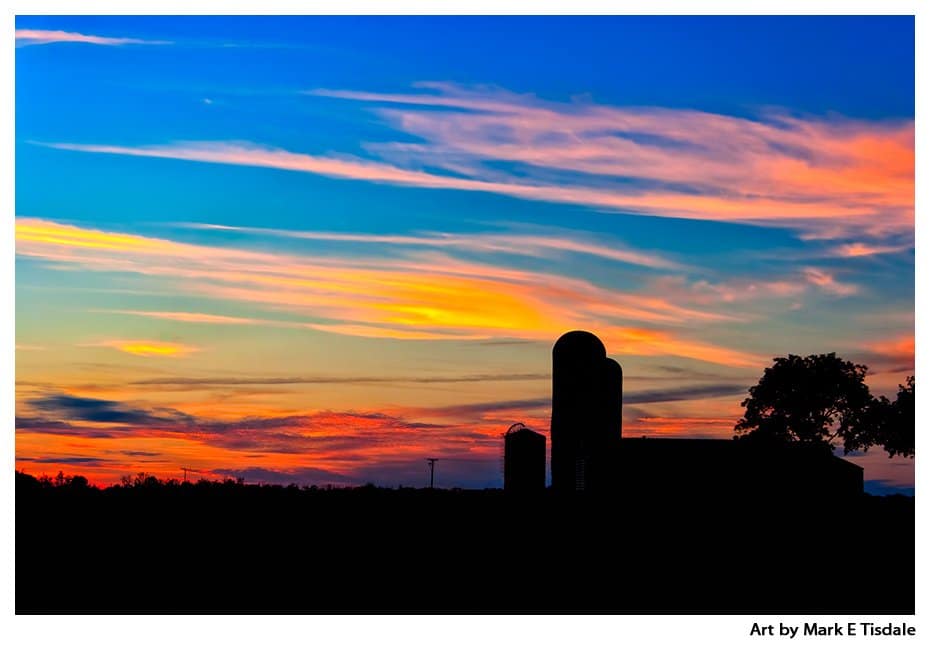This exterior landscape photo by Mark E. Tisdale captures a breathtaking sunset with a vibrant, blue sky adorned with wisps of white, gray, and richly pigmented orange and pink clouds. The horizon is aglow with an intense orange-peach light, creating a stark contrast against the sky. Silhouetted against this dramatic backdrop are three tall grain silos, possibly a farmhouse or barn, and two distant trees on the left, their dark outlines adding depth and moodiness to the scene. At the bottom of the image, a white background bears the inscription "art by Mark E. Tisdale" in black on the bottom right corner.